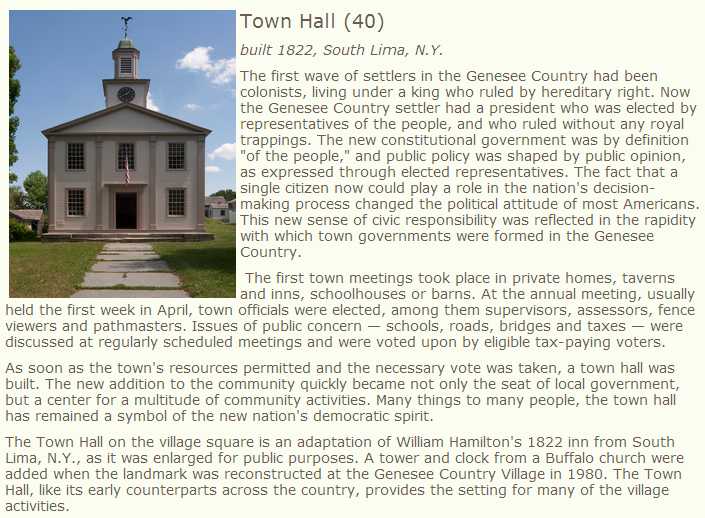The image shows a historic white town hall building, characteristic of early 19th-century architecture, with two stories and a weather vane crowning its roof. Situated in South Lima, New York, this town hall, built in 1822 as an adaptation of William Hamilton's inn from the same year, rests against a picturesque backdrop of a blue sky dotted with white clouds. It features an old stone walkway leading directly to its entrance, flanked by grass on either side, and an American flag prominently displayed near the front. The article adjacent to the image is set against a light background with dark gray text, detailing the building's historical significance and its role in the first town meetings of the area. The text also provides insight into the early settlers of Genesee County and the transition from colonial rule to a representative democracy. This town hall now stands as a testament to the region's rich heritage and community spirit.